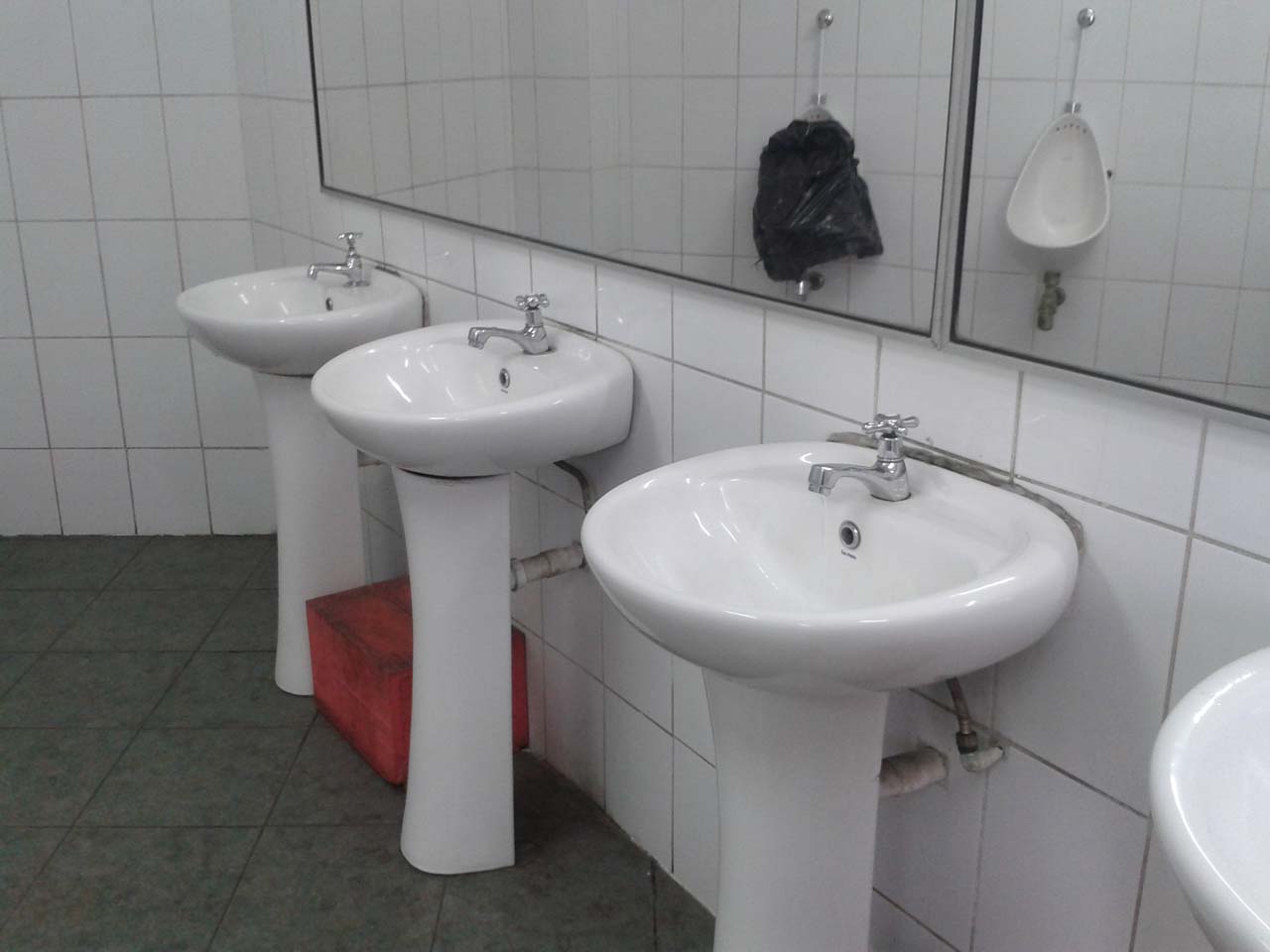This photograph captures the interior of a public men's bathroom, showcasing its detailed elements. The walls are lined with white tiles featuring dark gray grout, while the floor is adorned with dark gray tiles outlined by black grout. Positioned on the wall are two large mirrors, reflecting various bathroom fixtures. On the right side, the mirrors reveal two urinals; the one on the left is out of order, distinguished by a black trash bag covering it, whereas the one on the right is fully functional, displaying its silver flushing apparatus and drainage holes. Central to the image are four pedestal sinks, though the fourth sink is partially cut off due to the photograph’s framing. Each sink is white and fitted with a silver faucet with flower-shaped handles. Notably, a small red cube sits on the floor between the third and fourth sinks. The angled shot of the photograph provides a comprehensive view of these elements, converging into a detailed depiction of the bathroom's structure and fixtures.